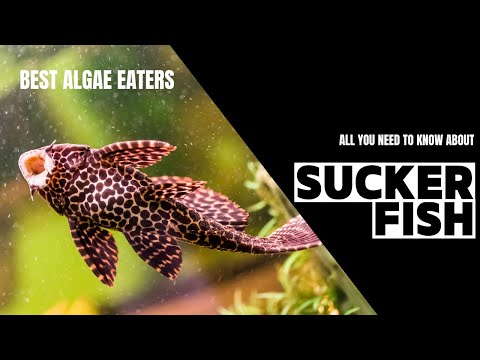The image appears to be an informational poster or book cover centered around suckerfish. It features a predominantly black background. The left side showcases a photograph of a suckerfish with a suction cup-like mouth open, likely attached to a fish tank's glass. The fish has a light gray body with distinctive dark spots and multiple fins arranged below its head. Above this image, white text reads "Best Algae Eaters." To the right, small white letters against the black background say, "all you need to know about," followed by "suckerfish" in large black letters on a white background. The layout is slightly horizontal, with a yellowish tint visible at the bottom right of the image.